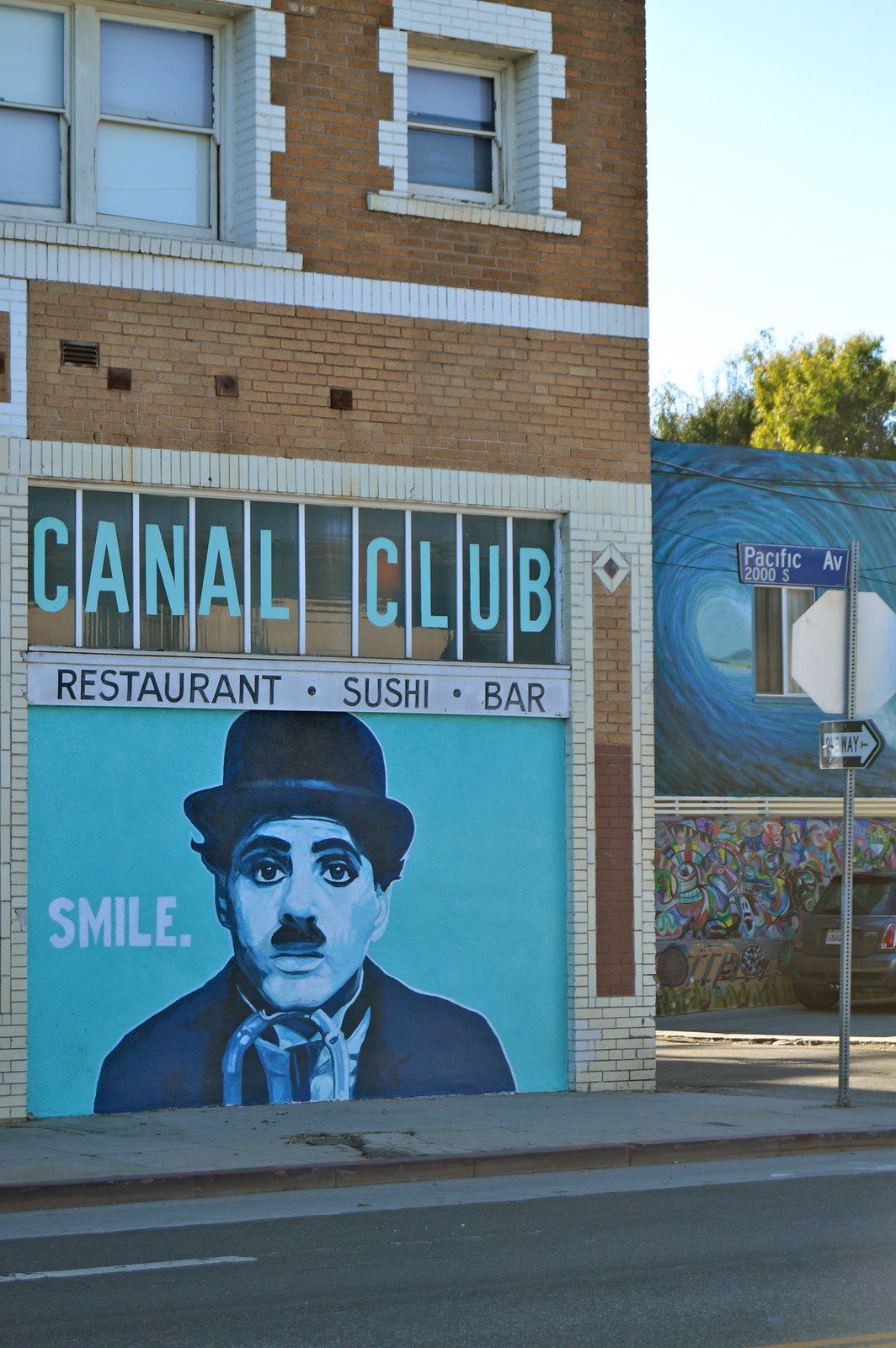This photograph features the vibrant corner of a brick building adorned with a striking mural. The mural, prominently displayed on the brown and tan brick wall, features a highly realistic painting of Charlie Chaplin in his signature derby hat, gazing forward with the word "SMILE" in bold white letters beside him. Above Chaplin, "Canal Club Restaurant Sushi Bar" is displayed across two sections: "RESTURANT SUSHI BAR" in black text on a white background, and "CANAL CLUB" in uppercase light blue lettering above the small windows on the second floor. In the foreground, a sidewalk runs along the base of the building, meeting a street marked by a street sign for Pacific Avenue with a one-way arrow. The clear blue sky and a portion of a tree can be seen in the top right corner, adding a touch of nature to this urban scene.